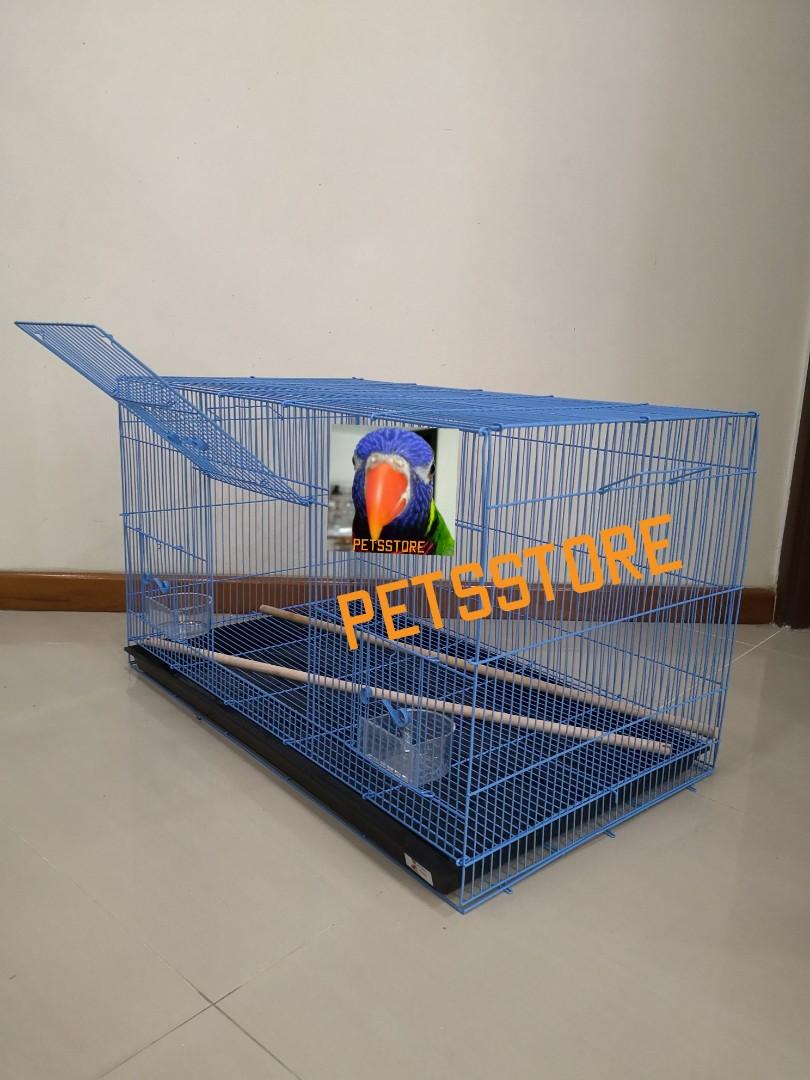The image features a medium blue rectangular cage positioned at an angle towards the 11 o'clock direction. The cage, with its black base and open door, houses two wooden dowels diagonally inside. It is set on a cream-colored floor composed of off-white diamond-shaped tiles. The background includes an off-white wall with medium wood baseboards running along the bottom. Superimposed in front of the cage, there is a vibrant headshot of a parrot showcasing a yellow-orange beak, purple head feathers, green shoulders, and grayish light trim around its white-gray eyes. Across the middle of the image, overlaid text spells "Pets Store" in a distinctive yellow-orange hue.